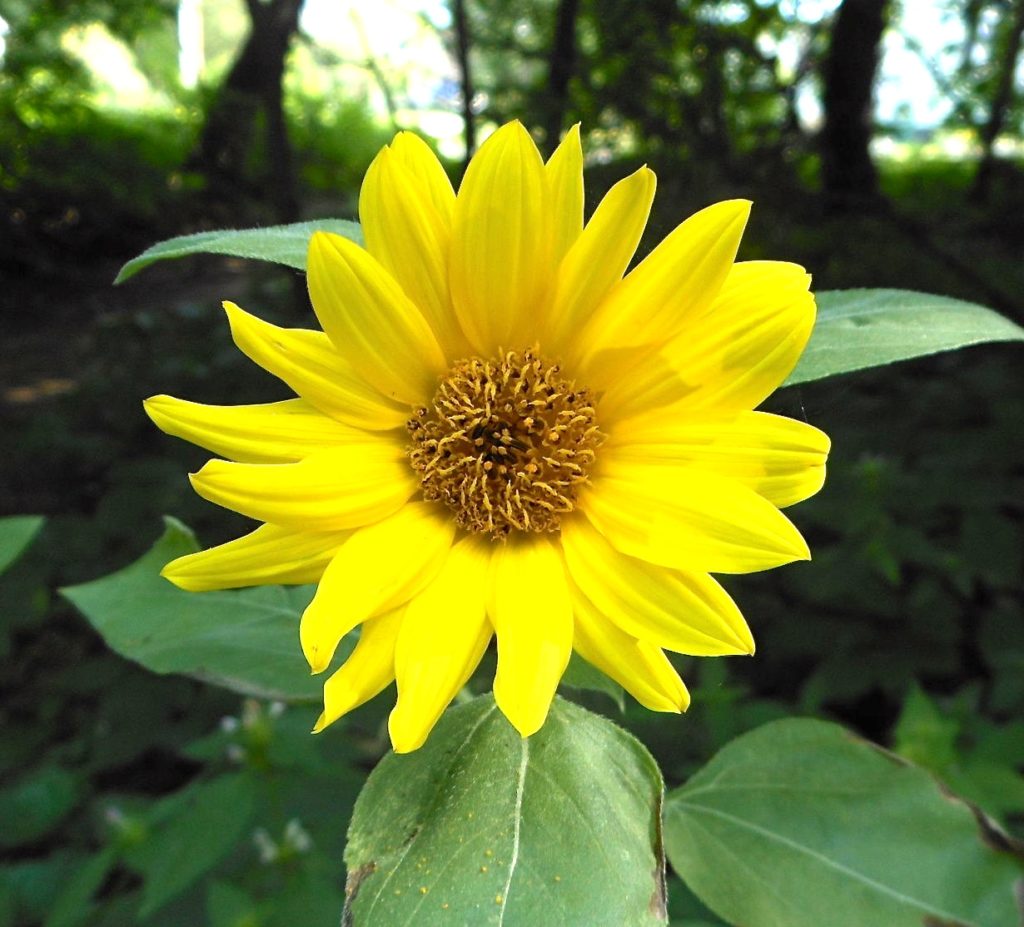The photograph is a full-color, close-up image of a fully bloomed, bright yellow flower, facing the camera directly and taking up most of the frame. The flower's numerous petals radiate around a darker yellow center disk, speckled with black. Surrounding the flower are small, green leaves with some brown spots and yellow speckles that appear to be pollen. A prominent broad leaf below the flower also has visible white veins and speckles. The background, which is blurred to emphasize the flower, reveals dense foliage with various shades of green, brown, and yellow, typical of a forested environment. Sunlight filters through the trees, creating a natural light effect that highlights the vibrant colors of the vegetation. The image captures the essence of a serene outdoor scene, with the focus sharply on the yellow flower and its immediate surroundings.